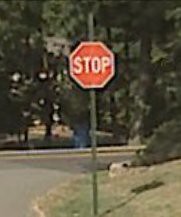The photograph showcases a classic octagonal red stop sign with white lettering, bordered in white. The stop sign is affixed to a thin green pole that stands several feet tall, situated in a small grassy area to the right of a roadway. To the left of the grassy strip, the road curves around, indicating where drivers should stop. The grass appears to be light green, possibly dried in patches. Behind the stop sign, a sidewalk or curb can be seen. The background is filled with tall, dark trees and some greenish pine trees, adding depth to the scene. The focus remains on the stop sign, which stands prominently against the natural backdrop and the road it regulates.